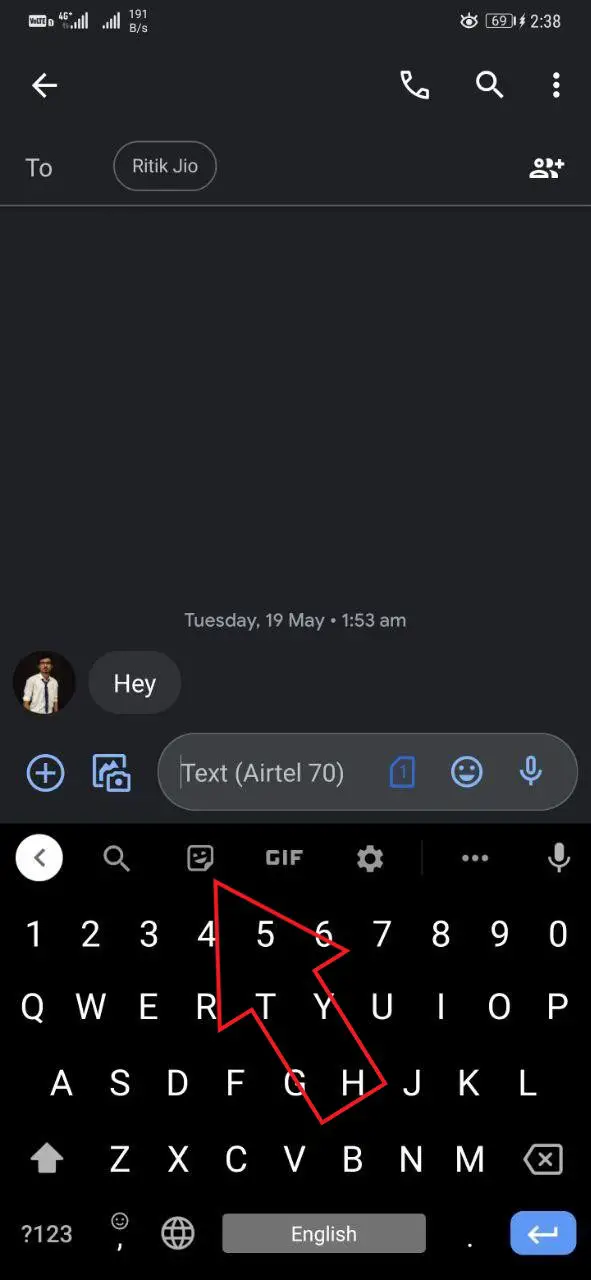The image depicts a text messaging interface on an Android phone. In the top left corner, various status symbols are visible, including '4G' and a reception icon. On the top right, there is an eye icon next to a battery indicator showing '69%' and the time '2:38'. Below this, on the left, a white arrow points leftwards, and on the right, there are icons for a phone, a magnifying glass, and a menu represented by three dots and a line.

Underneath, there's a section starting with a label '2', accompanied by an oval containing 'Riddick Geo'. This section seems to denote the messaging thread, though it's currently blank underneath. 

Further down, there's a timestamp 'Tuesday, 19th May, 1:53 a.m.' followed by a message bubble with the simple text 'Hey'. To the left of this message, there is a profile picture showing a person in a white shirt and tie.

At the bottom, within the text input area, there's a placeholder text 'Text Airtel 70' along with several icons: a blue '+' symbol, an emoji symbol, and a microphone symbol. Below this input area, the keyboard is displayed, indicating the QWERTY layout with English language settings. Additional keys include a globe icon for language switching and a blue send button with an arrow. There's also a prominent red arrow pointing towards an emoji icon, likely highlighting its importance or suggesting to use it.